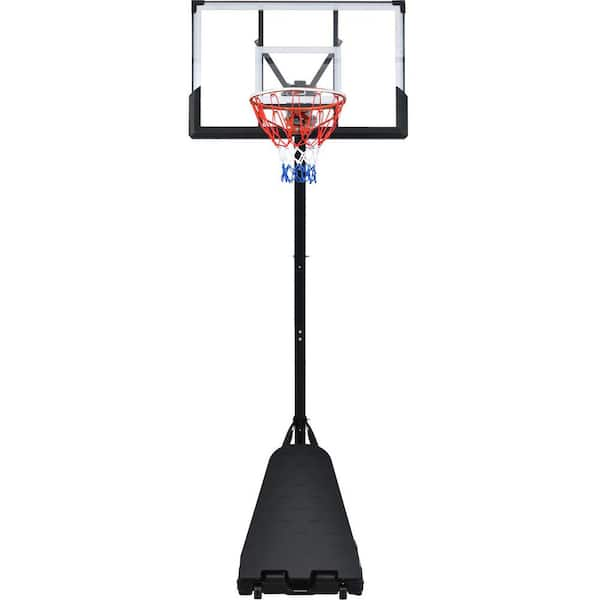This is a photograph of a portable basketball goal set against a white background, possibly cut out from its original image. The goal has a sturdy, black triangular base equipped with two wheels, designed to be filled with water or sand for stability and mobility. A tall, adjustable black metal pole extends from the base, featuring click-in extension dots. This pole supports a clear, rectangular backboard, bordered in black and white, which offers a transparent view of its mounting structure. Affixed to the backboard is a hoop with a red, white, and blue net, with the colors arranged from top to bottom in that order. The net's predominant color is red, followed by white, and finally blue at the bottom. The hoop is positioned within a smaller, horizontally mounted rectangle on the backboard, creating a well-balanced and functional design for a recreational or practice setting.